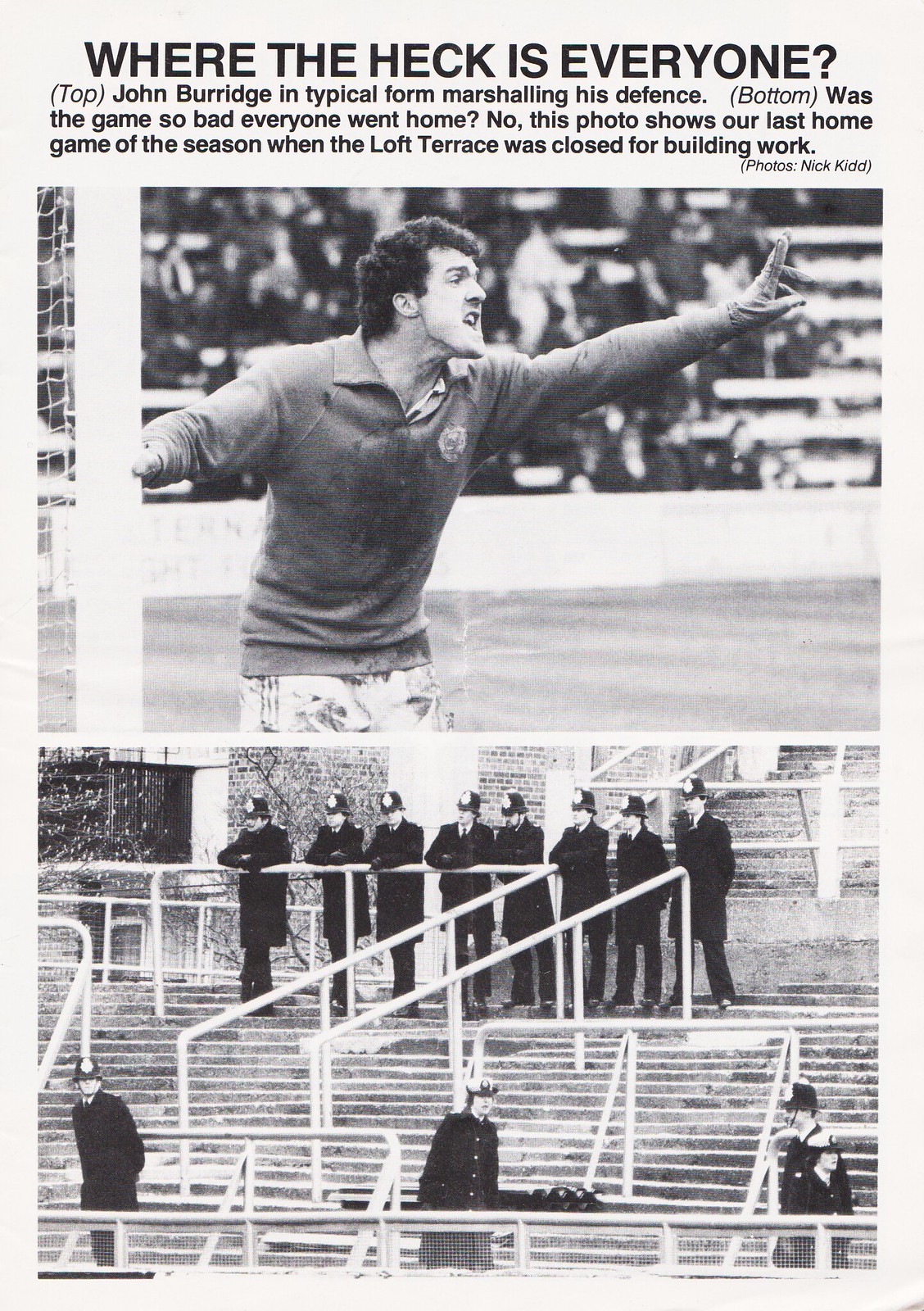A black-and-white magazine page features two photographs underneath a bold title, "Where the heck is everybody?" The top picture captures John Burridge, a soccer player, in action. He stands on a sports field, wearing a light-colored, collared rugby-style shirt and shorts. With his arm outstretched, his fingers raised, and his mouth open, he appears to be shouting, possibly directing his defense. The caption reads: "Top: John Burridge in typical form marshalling his defense."

The bottom photograph, labeled "Bottom: Was the game so bad everyone went home?" shows an empty set of bleachers from a recent season's last home game, with the caption clarifying, "No, this photo shows our last home game of the season when the loft terrace was closed for building work." The image features several uniformed security guards standing in rows, reinforcing the deserted atmosphere due to construction, not lack of attendance. The page, subtly aged to show wear, encapsulates a distinctive moment in the team's history through these evocative images and accompanying text.